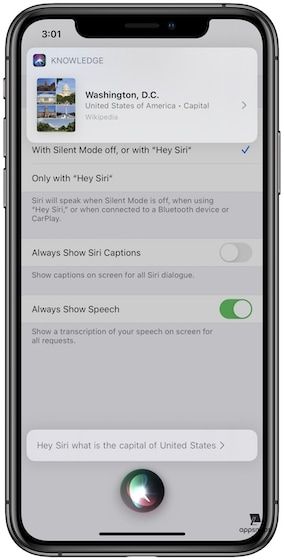The image captures a screenshot on a smartphone. The background is predominantly white. At the bottom of the screen, a text query is visible, reading, "Hey Siri, what is the capital of the United States?" in black font against the white background. Below the text, there is a colorful Siri icon that features a gradient of black, red, green, purple, and white hues.

At the top of the screen, Siri's response is displayed under the category "Knowledge." The response states, "Washington, D.C. United States of America, capital Washington," accompanied by blurry images of Washington, D.C. on the left side.

Further below, a section of the Siri settings is shown:

- The first setting option, "With Silent Mode off or With 'Hey Siri'," has a blue checkmark on the right side, indicating it is selected.
- The second option, "Only with 'Hey Siri'," is not selected.

An informational note below these options reads: "Siri will speak when Silent Mode is off, when using 'Hey Siri,' or when connecting to a Bluetooth device or CarPlay."

Two toggle switches are also visible:

- "Always Show Siri Captions" – This switch is toggled off, meaning Siri captions are not displayed for all dialogue.
- "Always Show Speech" – This switch is toggled on, highlighted in green, indicating that transcriptions of spoken queries will be shown on the screen for all dialogue.